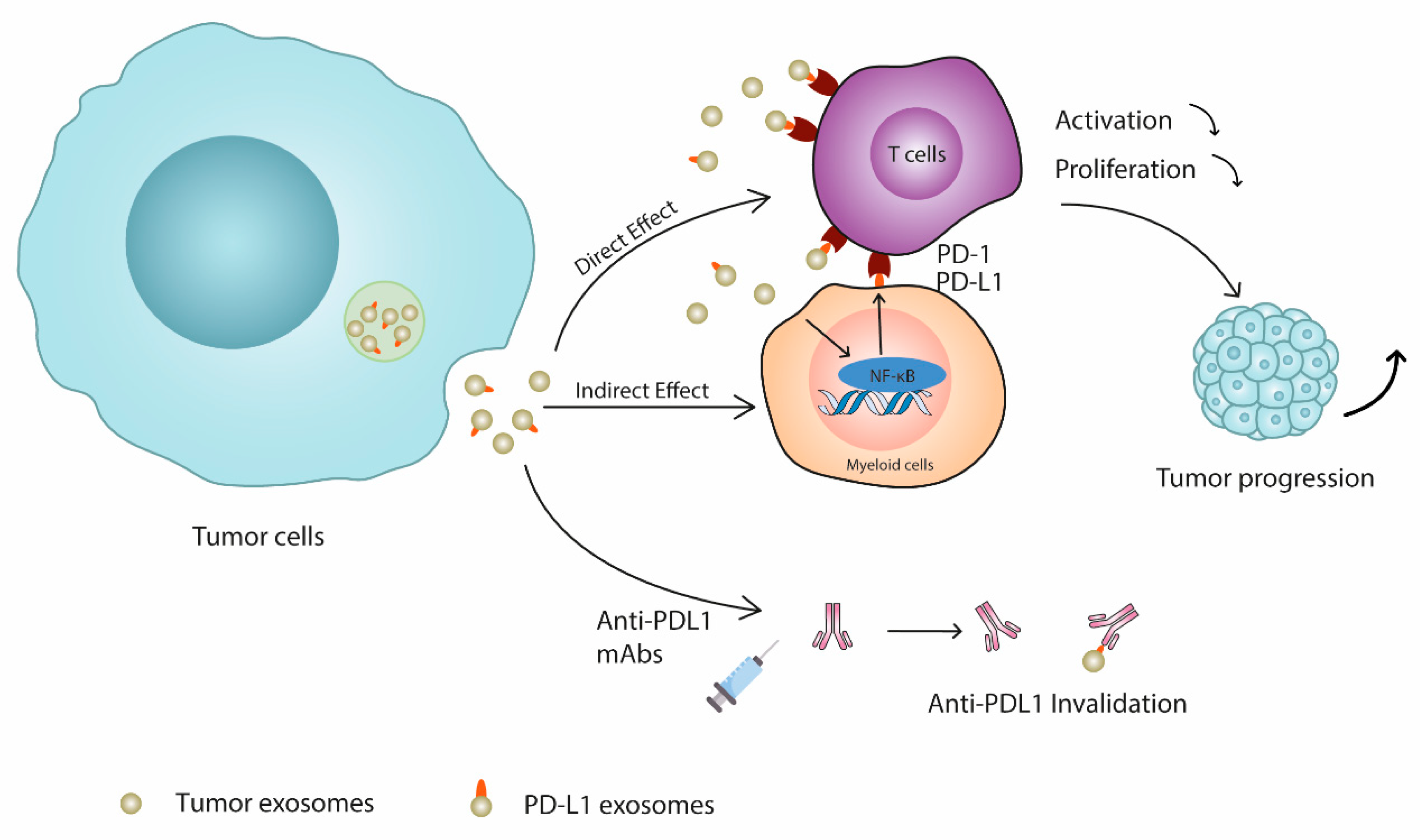This image is a detailed diagram depicting various cellular and molecular components involved in tumor cell progression. Predominantly, it features a blue, cloud-like figure on the left labeled "tumor cells." Inside this figure, there are darker blue circles and smaller olive-colored circles with red dots. To the right, there is another labeled section, displaying a light green circle housing additional smaller circles. Below this, "tumor cells" is written, indicating the corresponding shapes.

Further right, near the top, is a purple, rectangular object with rounded ends labeled "T cells," accompanied by another circular object labeled "myeloid cells," colored peach. Additional sub-diagrams show these cells and their interactions, with arrows illustrating pathways and effects such as "activation, proliferation," and "tumor progression." The diagram employs a palette of colors, including purple, white, light blue, pale yellow, black, darker blue, and reds to distinguish different elements and their functions.

The flow of information within the diagram is highlighted by arrows pointing to terms like "direct effect," "indirect effect," and "anti PD-L1 MABS," each leading to various outcomes like "activation proliferation" and "tumor progression." The entire setup distinctly portrays how tumor cells interact with different immune cell types and the potential outcomes of these interactions.